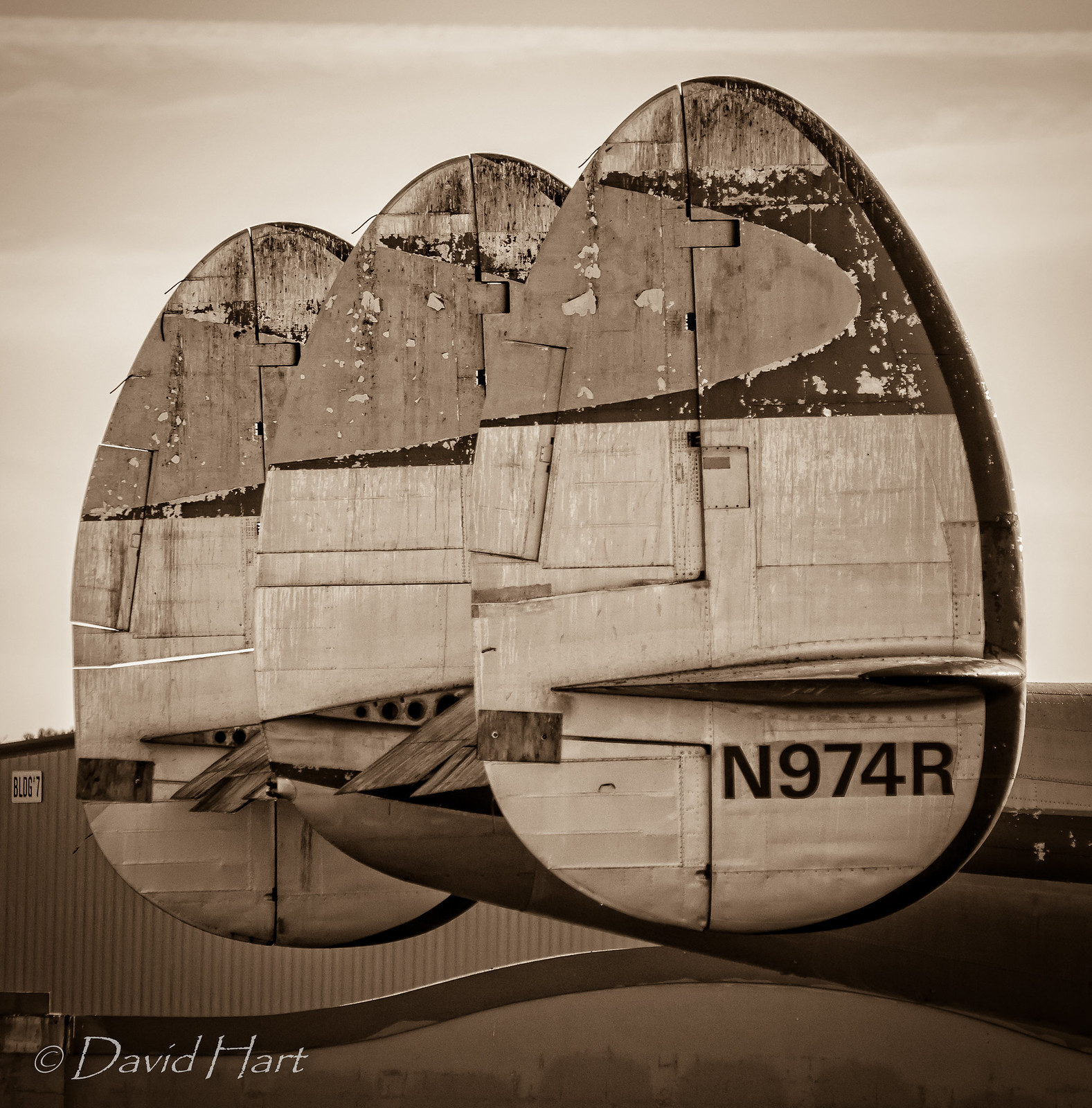This detailed sepia-toned art piece by David Hart features three distinct egg-shaped wooden forms that appear to be crafted from door-like material. The wood exhibits a rich variety of shades ranging from light brown to black, with notable discoloration and intricate detailing. Each egg-shaped piece is adorned with white specks, differing patches of wood, and a mysterious photograph-like element at the bottom that is somewhat difficult to discern. The central portion of the wood is light gray, adding to the composition's complexity. The backdrop is a sepia-toned outline of a building with metal siding and a black roof, imparting an almost surreal, nostalgic ambiance. In the background and foreground, a lighter sepia sky transitions to a darker brown ground. Notable markings include 'BL06-7' on the left side of the building and 'N974R' across one of the shapes. The piece concludes with a signature in white print at the bottom right: "copyright David Hart."